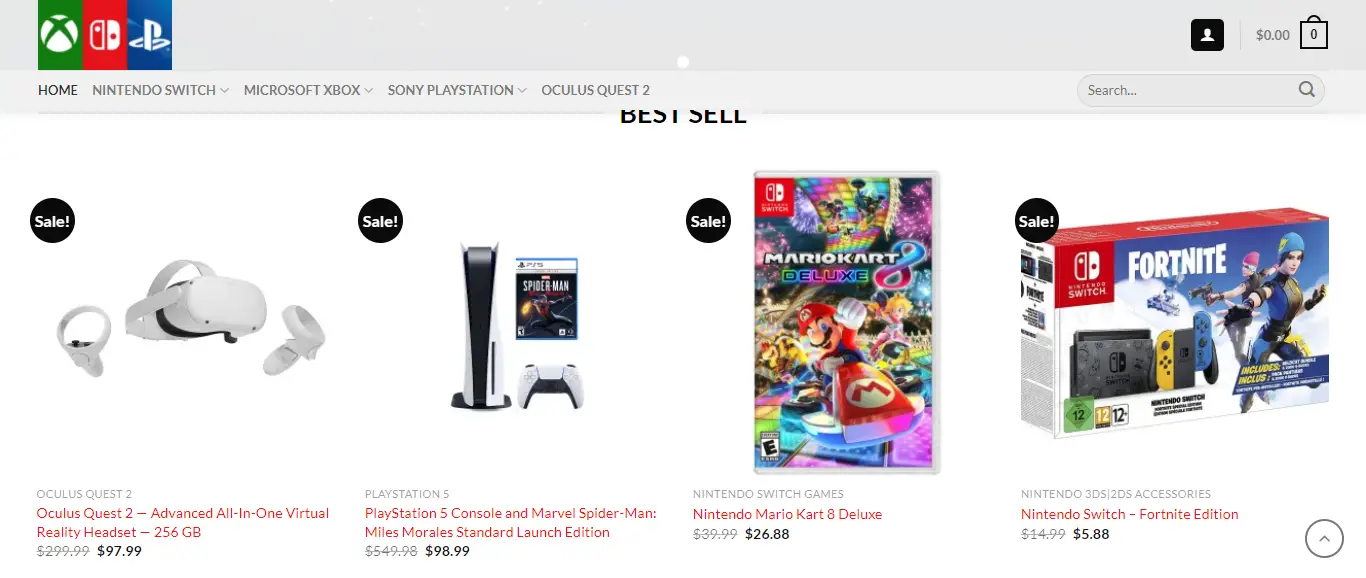The image showcases a layered display with different sections representing various gaming-related items. 

- The top layer is green, reminiscent of the Xbox brand, and is labeled as the internet switch.
- Below it, a blue section signifies the PlayStation brand.
- A black square with a person icon is also present, accompanied by text indicating "zero dollars," alongside a shopping bag icon, representing the home or internet switch for Microsoft Xbox and Sony PlayStation.
- The display features an Oculus Quest 2 headset, described as an "advanced all-in-one virtual headset" priced at $256, with a sale price of $97.99 also indicated.
- Additionally, it showcases a PlayStation 5 console featuring Marvel's Spider-Man, alongside mentions of "Marvel," "Saturn Legend," and a game titled "Mine Kart 8 Deluxe" priced at $26.88.
- Lastly, there's a Nintendo Switch Fortnite Edition box cover priced at $5.88, signifying the cost for this special edition console.